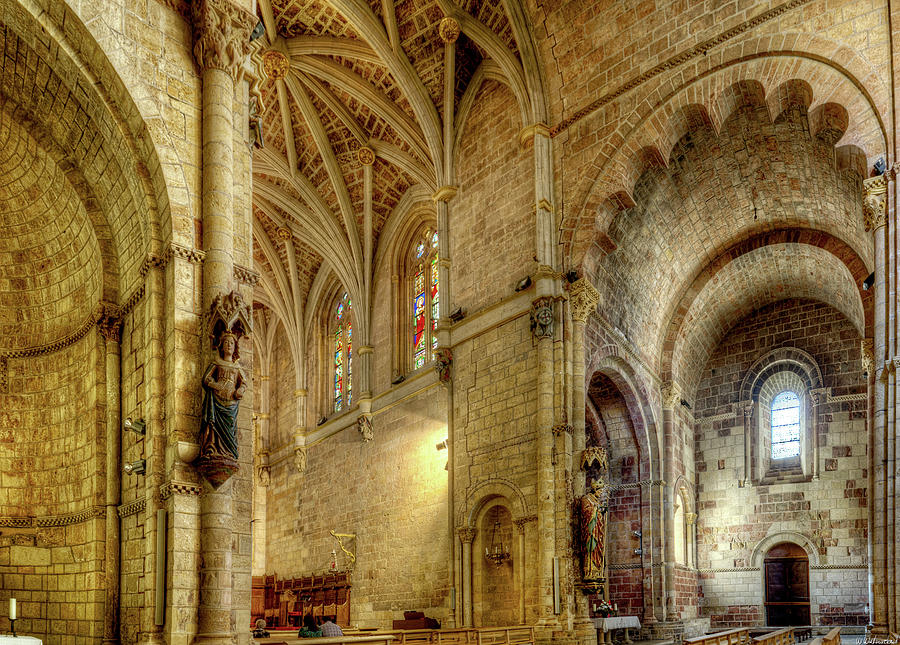This photograph captures the intricate interior of a large, medieval-style Catholic church. The architecture is dominated by tall, cathedral-like ceilings and expansive, arched structures, all crafted from a medium-toned stone or marble. The walls feature prominent pillars, each adorned with statues, likely of saints and possibly Jesus, emphasizing the church's spiritual and historical significance. The image highlights two notable areas of stained glass windows: one positioned under an arched ceiling to the right, and another set in the background above the pews. These windows display detailed religious designs in vibrant colors such as blue, red, green, white, and yellow, including depictions of a bird and various figures. In the foreground, a row of pews holds several people, possibly three, seated in quiet prayer, adding a serene, reverent atmosphere to the scene.